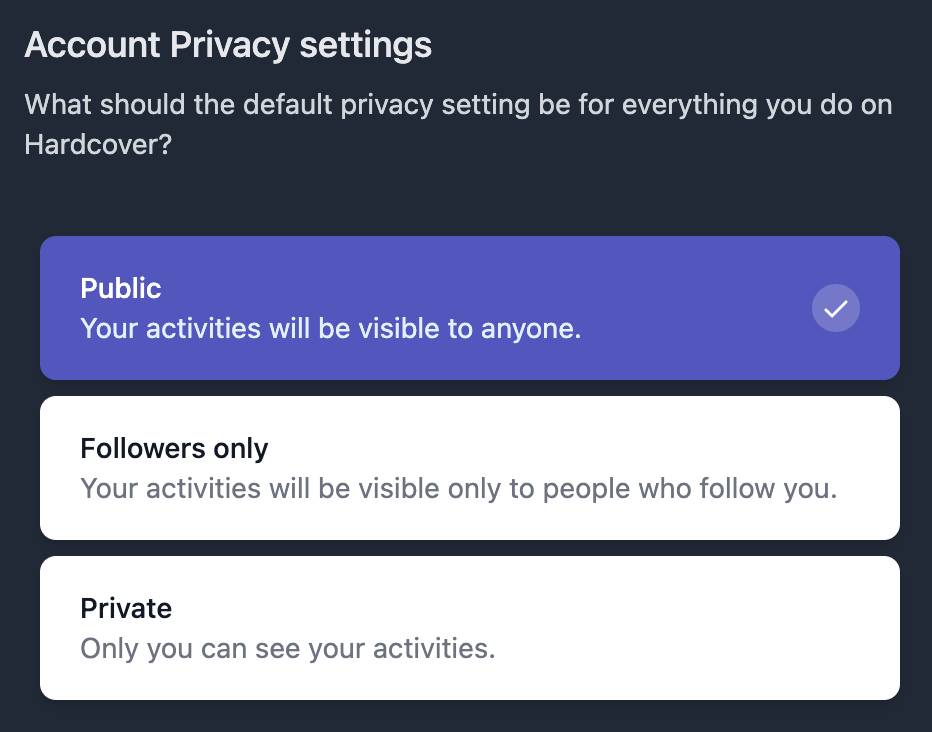Here is a more detailed and cleaned-up caption for the image described:

---

This is a detailed screenshot from the "Hardcover" app displaying the "Account Privacy Settings" section. The app interface features a sleek black background with prominent white text. At the top, the heading reads "What should the default privacy setting be for everything you do in Hardcover?" Below this, there are three distinct rectangular options that the user can select to set their account privacy settings.

The first option, "Public," is highlighted in a blue box with white text, indicating it is the current selection made by the user. Its description states, "Your activities will be visible to anyone." 

The other two options, "Followers Only" and "Private," are presented in white boxes with black and grey text. The "Followers Only" option specifies that "Your activities will be visible only to people who follow you." The "Private" option notes that "Only you can see your activities."

This screenshot effectively captures the user interface designed to provide users with clear choices regarding their privacy settings within the Hardcover app. The user in this instance has selected "Public" as their preferred setting.

---